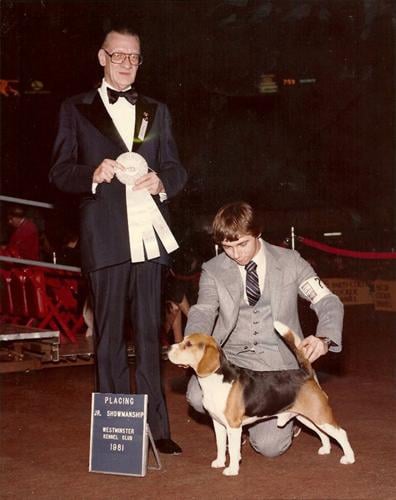In the photograph of a dog competition, the scene is set in a dimly-lit arena. On the right side of the image, a young man dressed in a well-fitted gray suit, vest, and tie, is kneeling down, carefully positioning a beagle by holding its nose and tail up. An armband on his sleeve displays the number seven. Next to him, on the left, stands an older gentleman in an ill-fitting dark suit and bow tie, wearing glasses and holding an award ribbon. The older man is facing the camera directly. The background shows a sign partially reading "Westminster Kennel Club 1981," suggesting that this event dates back to 1981. The colors in the image include a mix of grays, blacks, browns, reds, and beiges. There is no visible audience, making the focus solely on the young handler, the beagle, and the award presenter.